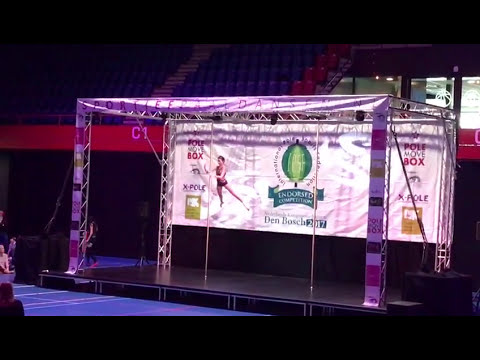The image depicts a stage set up inside a gym arena, evident from the seating arrangement in the backdrop. The stage itself is a pop-up structure with metal supports and a large black platform. A banner runs along the front supports and over the top, though it has some sections with folded-over material obscuring parts of the text. The backdrop prominently features a wide white banner displaying a large green logo in the center with the text "Den Bosch 2017" underneath it. Additionally, there's an image of a dancer on the left side of the banner and phrases such as "International Health Federation" and "endorsed competition" are visible. There are minimal people present, with a few individuals seen on the outskirts in the bottom left corner. The setup seems to be for a health or fitness competition, possibly involving some form of gymnastics or pole dance performance, as suggested by references to “pole move box” and “X pole” on the banner.